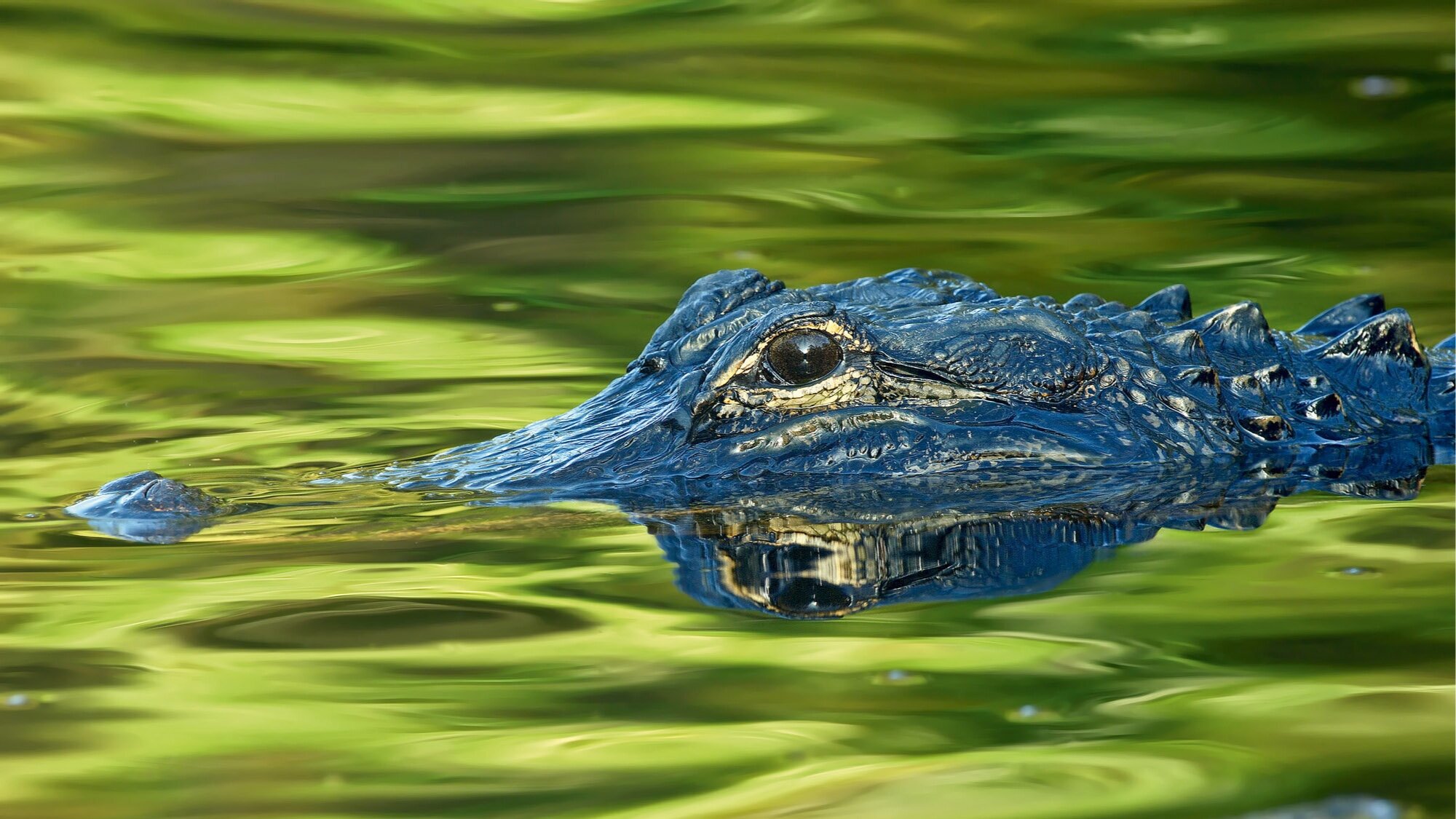This detailed photograph captures the profile of a crocodile's head emerging from a greenish pond. The crocodile's scaly head, part of its back, snout, and neck are visible as it moves from the left to the right side of the frame. The brightly colored image features a soft-focus watery background that appears altered, giving it a blurred, abstract look. The crocodile, with a large, dark black eye that directly meets the viewer's gaze, dominates the center of the image. The eye's reflection shimmers in the water below. The skin of the crocodile displays a bumpy, textured appearance with bluish and brownish tints, and there are distinct ridges along its neck. The photo captures the stillness of the moment, with the crocodile appearing to glide silently, perhaps hunting in its natural habitat, with no other distractions or text in the image.